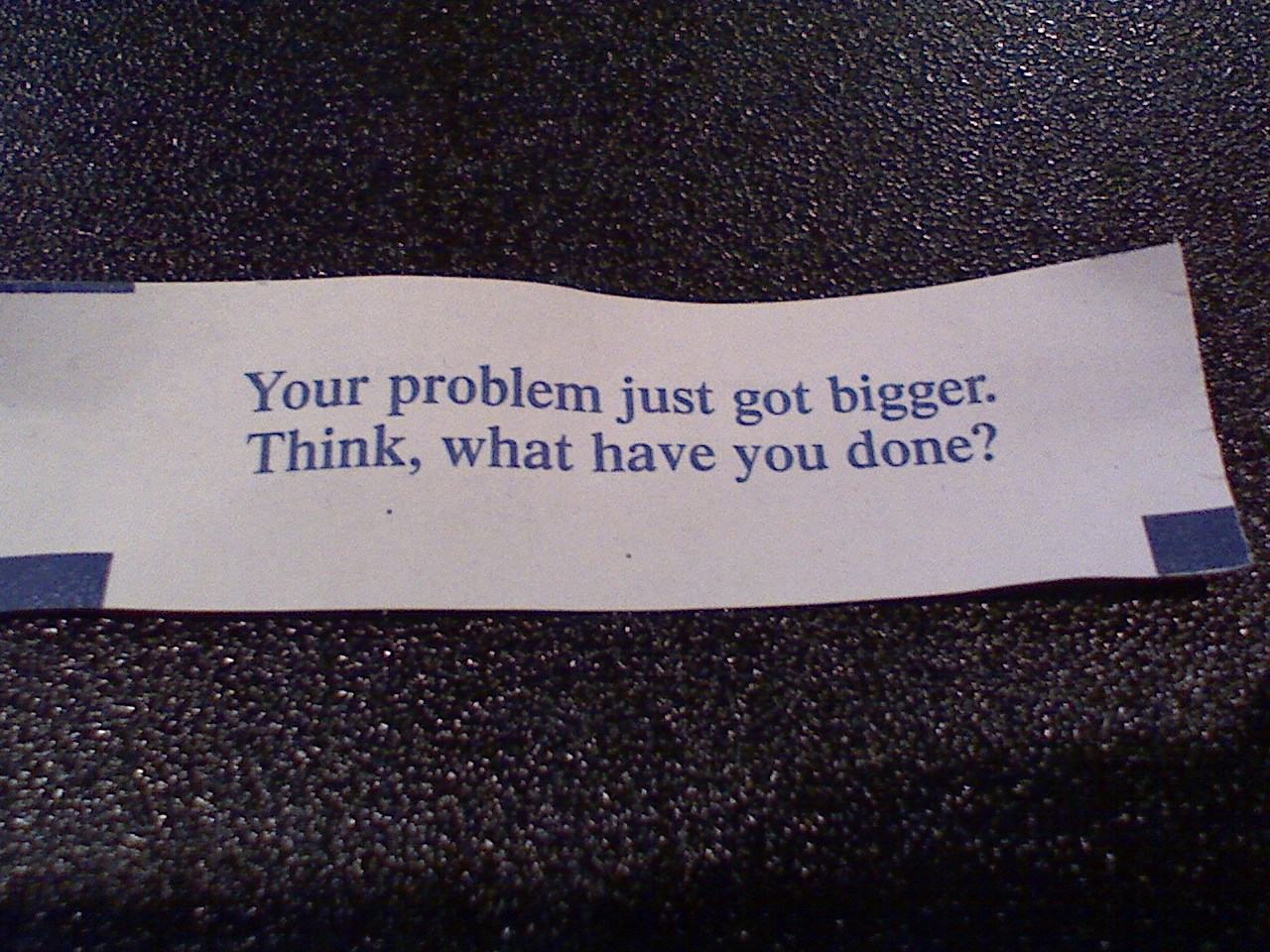A close-up image showcases a fortune cookie slip placed on a grain-textured, black tabletop speckled with white. The paper is mostly white with blue lettering, arranged in two lines that read, "Your problem just got bigger. Think, what have you done?" The fortune slip, rectangular in shape, has small blue boxes in three corners, missing only in the top right. The lighting highlights the white speckles on the dark surface, giving a contrasting backdrop that focuses attention on the fortune's ominous message.